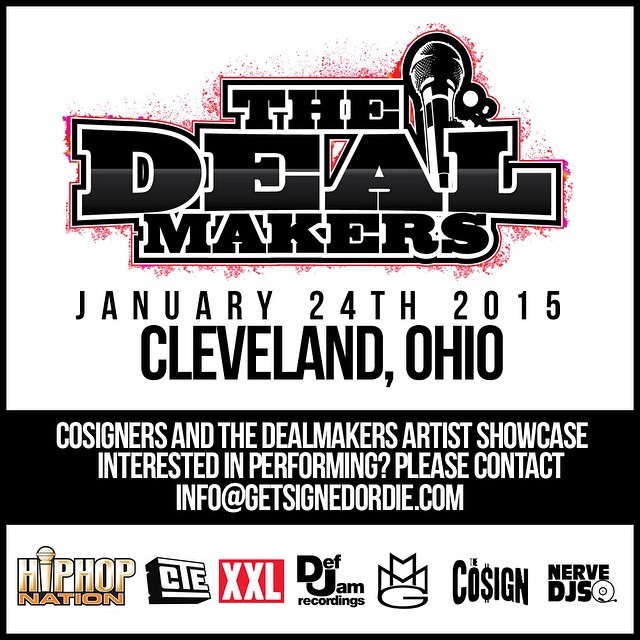This visually striking event flyer announces "The Dealmakers" with bold, oversized text on a white background, highlighted by a microphone icon within the letters "A" and "L." The title, "The Deal Makers," is accentuated with red splatters, adding a dynamic, almost electric effect. Directly beneath, it details the event date and location: January 24th, 2015, in Cleveland, Ohio.

A black strip below the main title features white text inviting artists to perform at "Co-signers and The Deal Makers Artist Showcase." It includes a call to action: "Interested in performing? Please contact info@GetSignedDone.com."

The lower section of the flyer, set on a white background with black and red print, showcases a series of iconic brand logos such as Hip Hop Nation, CTE, XXL (in red), Def Jam Recordings, MMG, Co-sign, and Nerve DJs, solidifying the event's emphasis on hip-hop culture and its prestigious affiliations.